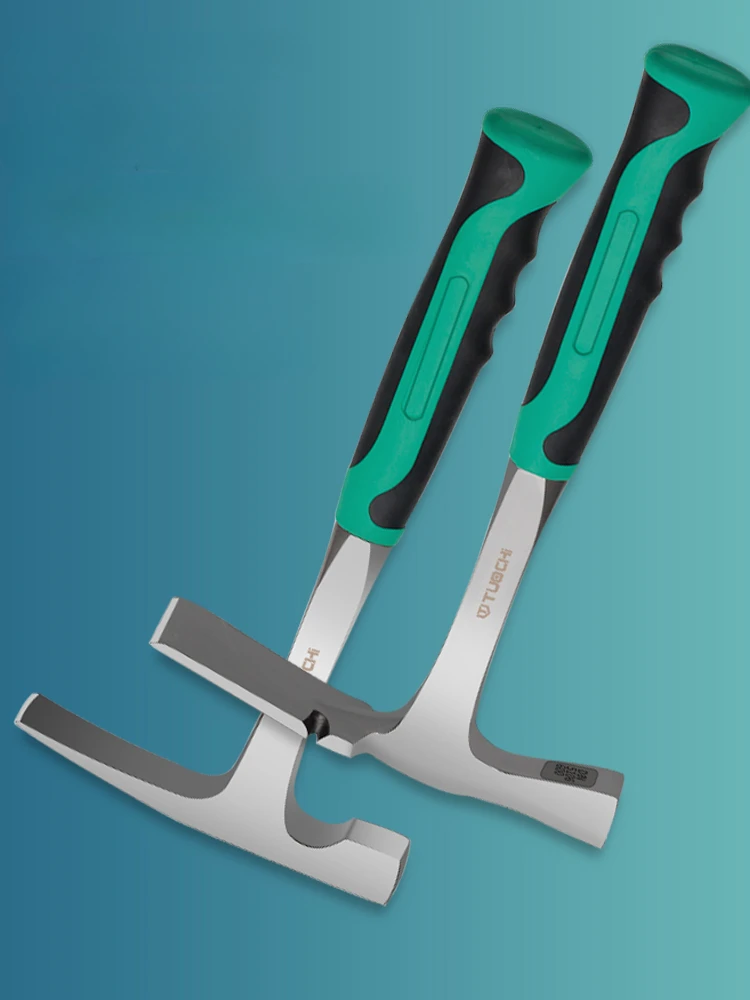The image features two nearly identical hammers placed in an inverted, overlapping fashion on a turquoise background. Both hammers have metal heads, which are likely made of steel, and exhibit a grey or silver color. The handles of the hammers are positioned pointing toward the top right corner of the image while the metal heads point downwards to the bottom left. 

The handles feature a rubber grip that is primarily green with black accents along the sides. The turquoise background of the image fades from a darker shade on the left to a lighter shade on the right, providing a gradient effect. 

Text, likely the company name and possibly reading "Tushy," is inscribed in small font on the steel part of the hammer heads. Despite their similarities, there are slight differences between the two hammers: the hammer on the lower side has a small darker part on the T-shaped head and a dip on the right side, whereas the top hammer displays a larger grey area without the dip. The setting is distinctly styled to highlight the tools against the vibrant blue backdrop.